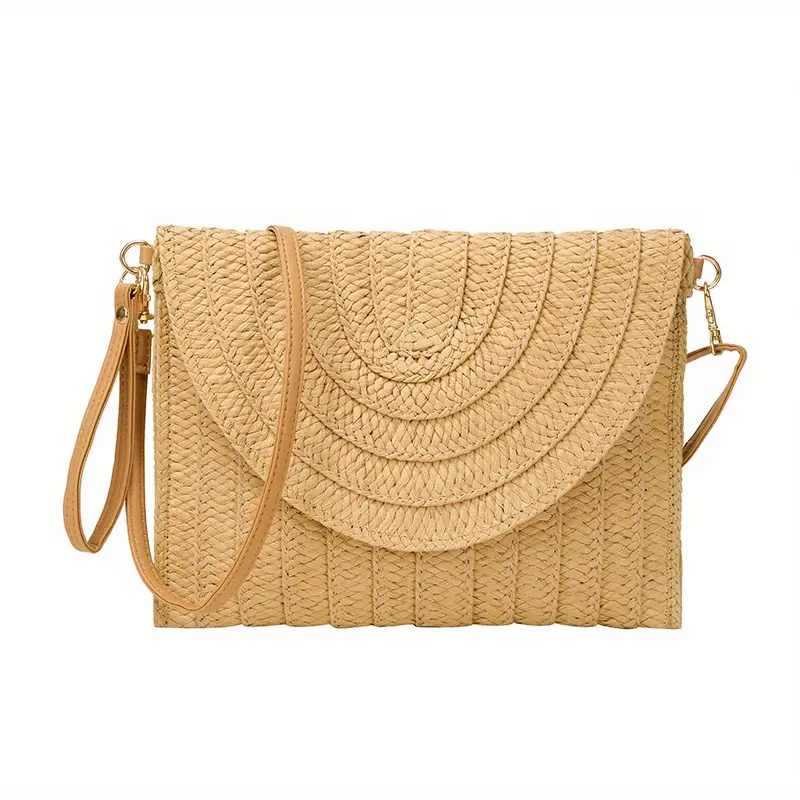This image showcases a boho-style handbag meticulously crafted from a natural fiber, giving it an earthy, handmade appearance. The handbag, woven in a beige-tan tweed, features a half-circle flap that faces forward. It is complemented by a darker brown leather strap, detailed with visible stitching. The strap is attached via small golden clasps to metal loops on either side. Additionally, there's a smaller wrist strap adorned with a gold rivet. The entire scene is set against a stark white background, highlighting the purse without any distractions. This straightforward presentation, likely intended for an online fashion retailer, emphasizes the handbag's rustic texture and intricate craftsmanship.